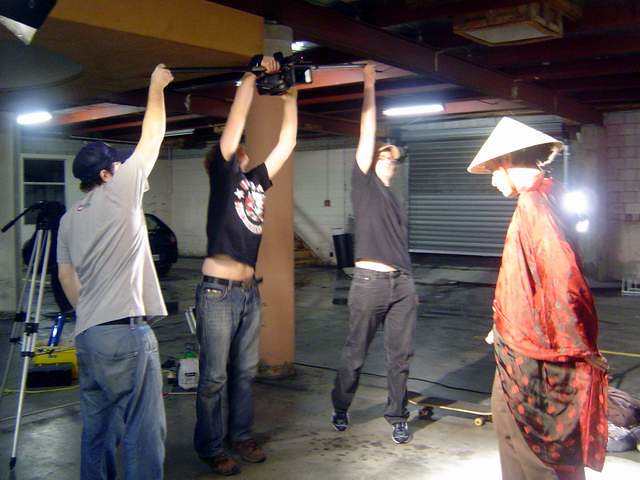This photograph captures a bustling scene, presumably a photography or film session, set within a spacious and somewhat dark warehouse or garage environment. Standing in the middle of the composition, an Asian individual dressed in a traditional geisha-like costume—red robe with black detailing and a triangular hat—appears to be the focal point. Surrounding this central figure are three young men, each dressed in casual attire of short-sleeved shirts and blue jeans, collectively engaged in a creative endeavor.

The man on the left, distinguishable by his blue baseball cap and gray shirt, holds an unidentified object, likely related to the photography or filming equipment. The man in the middle, dressed in a black shirt, extends his arms overhead, firmly grasping a camera or camcorder to capture the scene. The third man, positioned on the right, is equipped with what appears to be a lighting device or an accessory piece associated with the camcorder, his outfit matching the informal style of the other men with a dark gray shirt and black shoes.

The setting further highlights the industrial aesthetic, with details such as a silver roll-top garage door, extensive fluorescent lighting, and a concrete floor adding depth to the scene. Scattered around are various pieces of equipment, including a visible tripod and a skateboard on the floor, enhancing the impression of a dynamic and possibly improvised setup. The wooden roof structure and additional lighting elements suggest that this is a practical, working space dedicated to creative projects or might be a student's filming location.